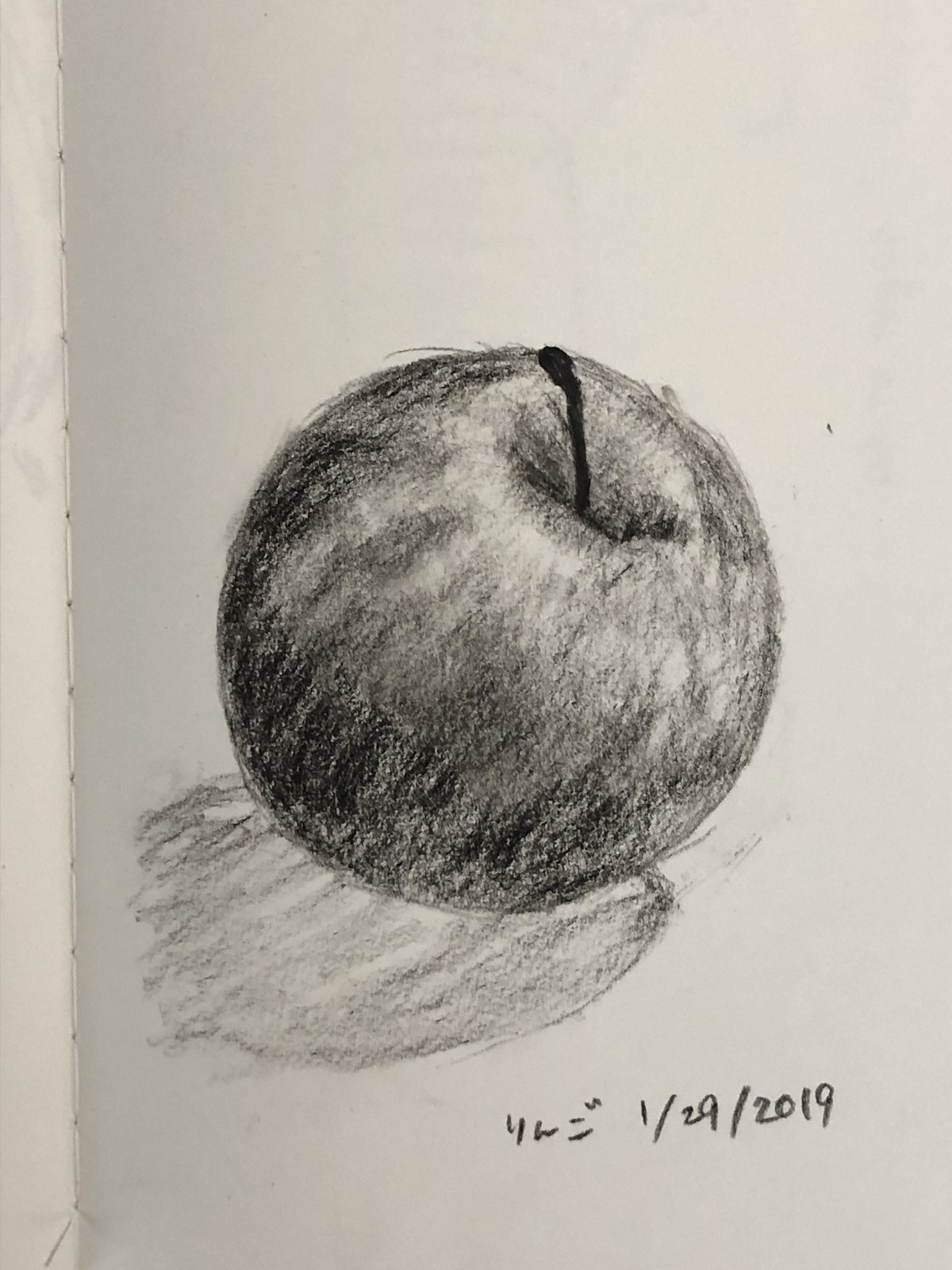This detailed charcoal-style drawing, rendered on an off-white sheet of paper with a visible crease along the left-hand side, appears to be from a notebook. The artwork features a meticulously shaded apple, emphasizing its round form. Darker shading marks the top indent from which a black stem emerges, creating a striking contrast. The apple's left side is heavily shaded, indicating the light source falls from the opposite direction. Below it, a circular, gray-toned shadow reflects the apple's form. The artist inscribed the date “1-29-2019” in the bottom right corner, likely marking the completion date of this intricate piece.